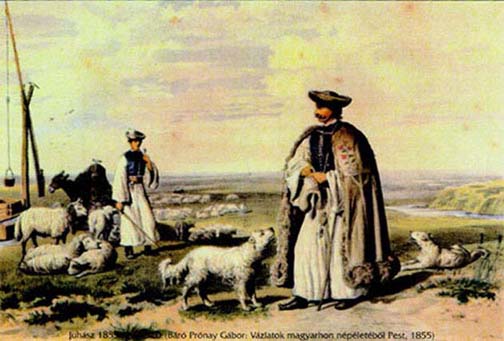The image depicts an intricate, multi-colored outdoor painting set in natural light. Horizontally rectangular with no border, the artwork features faint black text at the bottom, barely legible and in a foreign script, alongside the date 1855. The setting appears to be a green field on a hill with splashes of tan soil. To the far right, a blue river snakes into the distance. In the foreground, two men, likely sheep herders or farmers, are central to the scene. One, positioned on the right, dons a flowing white robe and a tan cloak, possibly made of fur, with a white dog gazing up at him. The other man, slightly to the left and further back, wears a white robe, a blue vest, and a round hat, holding a long stick. Both are surrounded by a multitude of sheep, some standing and some resting. The sky is a vibrant mix of yellows, blues, purples, and whites, adding to the painting's dynamic color palette that includes shades of white, black, blue, tan, beige, and green. The attire suggests a period earlier than 1855, characterized by long gowns and traditional garments.